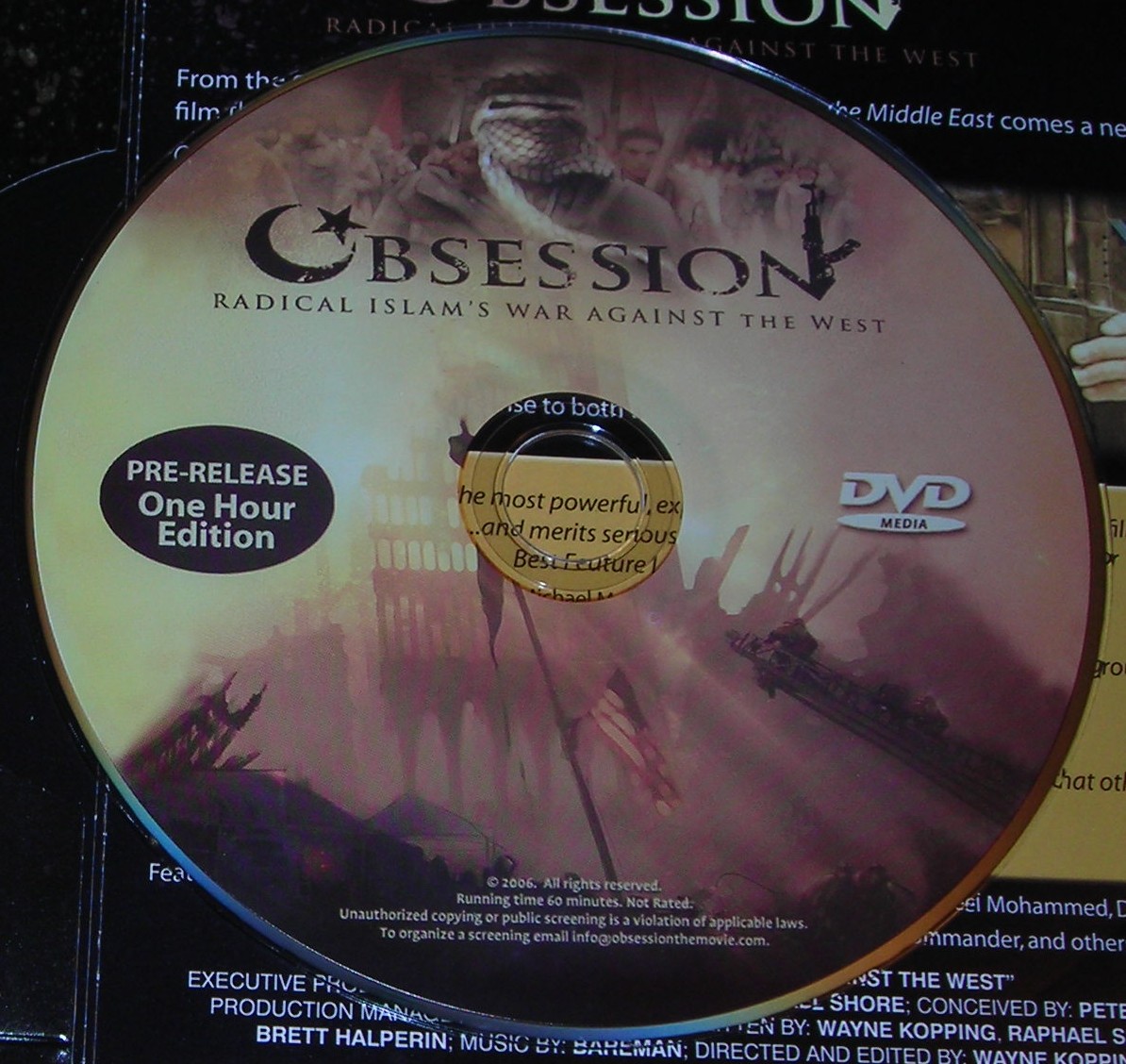This is a close-up image of a DVD. The DVD features a detailed background that likely corresponds to its case, filled with tan and darker hues. Prominently displayed at the top is a masked figure, whose face is almost entirely obscured by a white covering, suggesting Middle Eastern attire. This figure stands against a backdrop populated with indistinct figures, torn buildings, and American flags, hinting at a scene of conflict. The title of the DVD, "Obsession," is configured prominently, with the 'O' styled as a crescent moon cradling a star, and the 'N' incorporating a machine gun into its design. Subtitled beneath the main title are the words "Radical Islam's War Against the West." To the left of the central imagery, within a black oval, the words "Pre-Release, 1 Hour Edition" are written in white. On the right, it states "DVD Media." Additional text at the bottom specifies "Copyright 2006, All Rights Reserved," a running time of "60 minutes," and "Not Rated." It warns against unauthorized copying or public screening, directing those interested in organizing a screening to email info@ObsessionTheMovie.com.